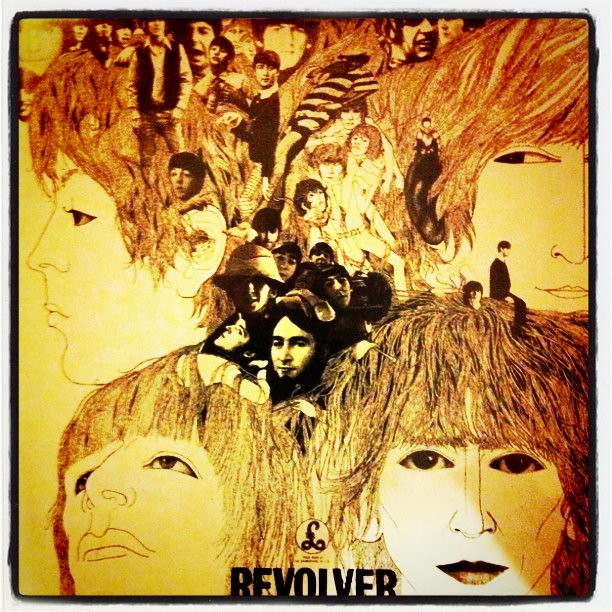The image is a detailed and artistically complex depiction, likely the LP cover for The Beatles' "Revolver" album. The overall tone of the image leans towards sepia, with a mixture of both detailed illustrations and photographic collages. It's presented in a square format with a black border. The background features a multitude of intricately drawn faces with long, messy hair and black, hollow eyes, set against realistic photographs. The faces are arranged in various directions. Four prominent faces are positioned near the corners, each looking outward. The center of the image contains a dense collection of these human faces and figures. At the bottom, in large black capital letters, the word "REVOLVER" is clearly visible. Above this text lies a white circle, within which is a curved L shape forming a loop resembling an infinity sign. Additionally, there are some darker, more realistic heads interspersed among the artistic drawings.